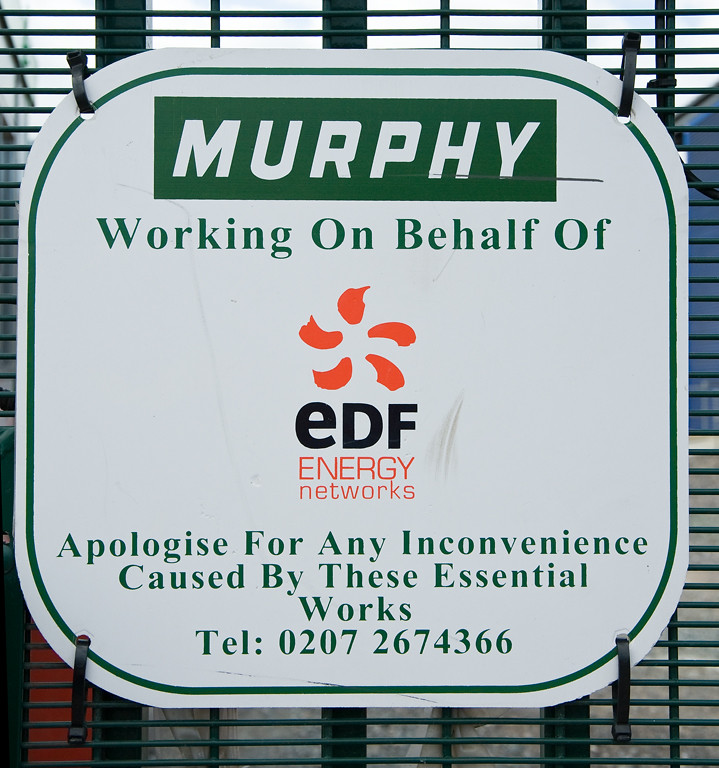The image features a white, rounded-corner sign secured with zip-ties to a tightly woven, dark green metal grate. The grate’s color complements the branding on the sign. The sign has a thin dark green border, and at the top, a dark green rectangle with white capital letters reads "MURPHY." Below this rectangle, green text against the white background states "working on behalf of" followed by a pink logo resembling a flower without a center, which represents EDF Energy Networks. Further down, green text continues with "apologize for any inconvenience caused by these essential works," and finally provides a contact number: 0207-267-4366.